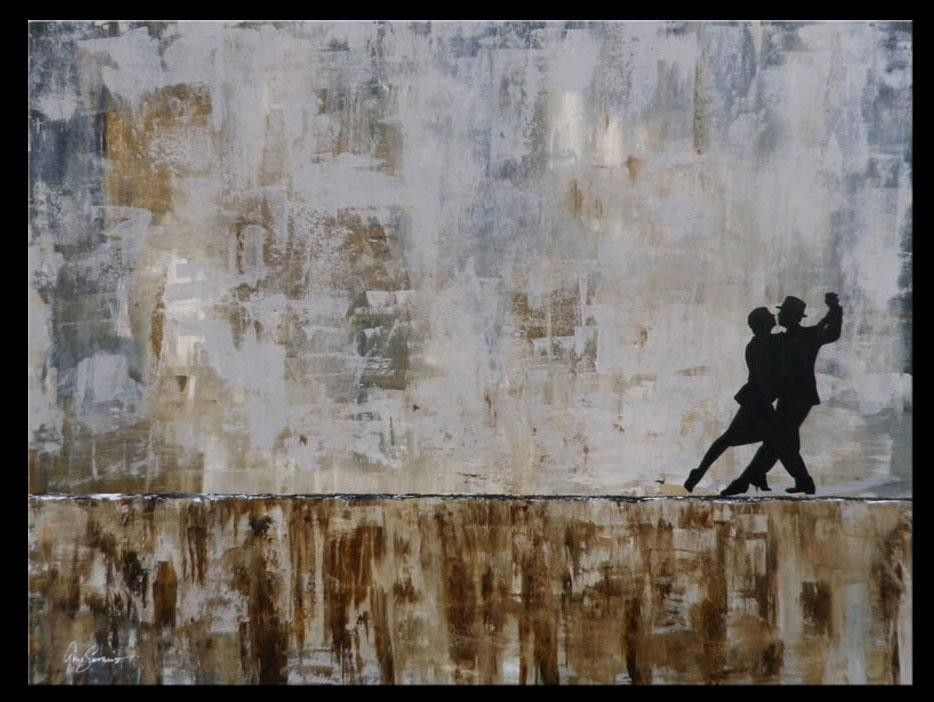The painting, surrounded by a narrow black frame, features a silhouetted couple dancing the tango. The man, who is wearing a brimmed hat, leans slightly back while the woman, dressed in a knee-length skirt, embraces him with her left leg extended gracefully backward. Mirroring her pose, the man's right leg is extended forward. The dancers' arms are held up in an L-shape. The background is a blend of smudged dark and light grays, rusty browns, and hints of blue, giving it an old-school graffiti or stonewashed appearance. A horizontal gray line about a quarter of the way up the canvas indicates the floor or stage, with darker brown brush strokes below suggesting texture. The overall palette of the painting is dominated by shades of brown, gray, and black, with no additional text or distractions, focusing entirely on the intimate dance of the silhouetted figures.